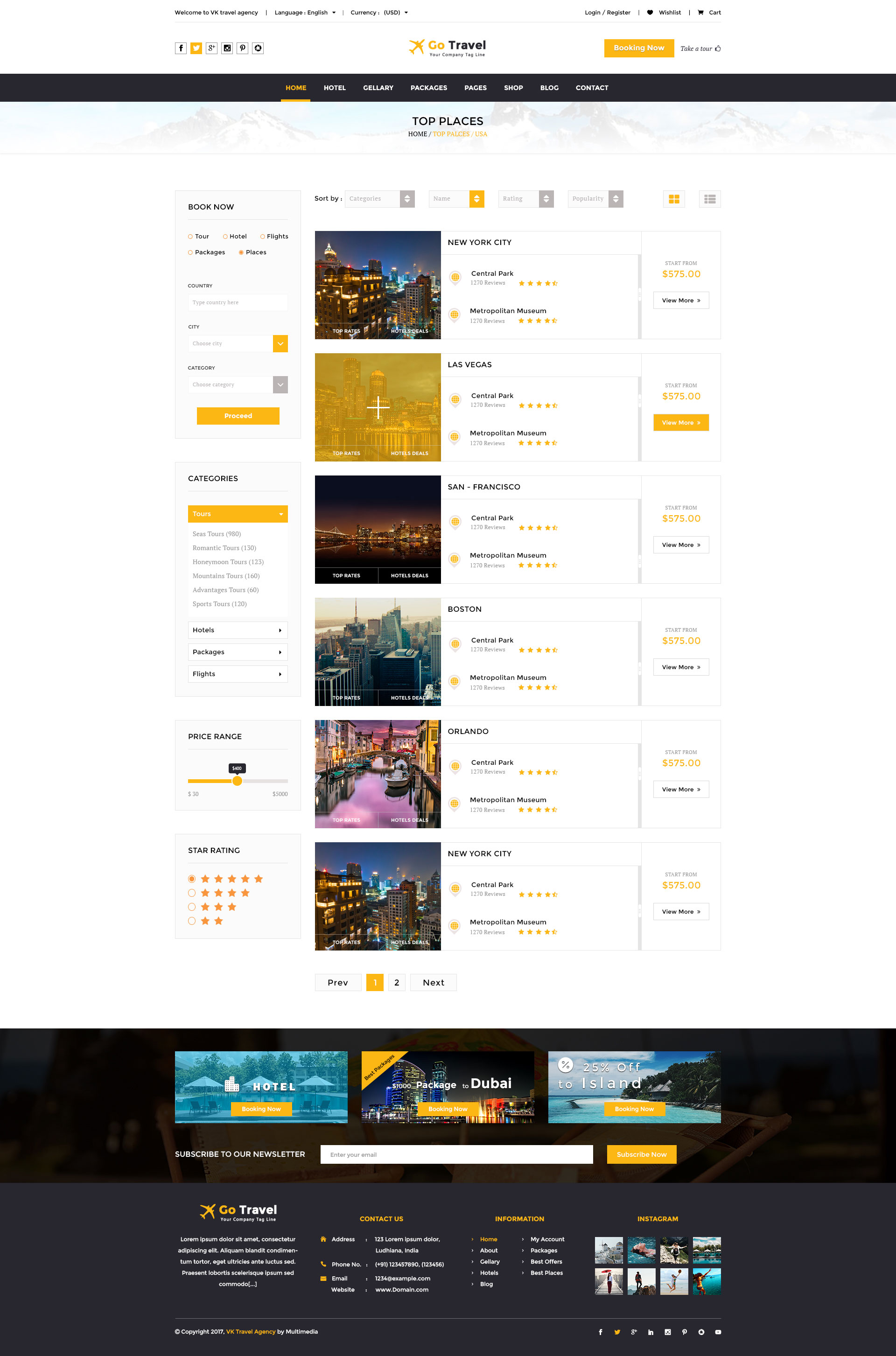This image is a screenshot of a travel booking website. The interface features a predominantly white background with a banner image situated behind one of the headers. The banner depicts a light, nearly transparent image of a snow-capped mountain range set against a blue sky. 

At the very top of the page, the website is branded as "Go Travel" accompanied by an icon of an airplane. The airplane silhouette and the word "go" are highlighted in yellow, while the word "travel" is in black. Beneath this, there is a black navigation bar containing seven to eight different tabs.

The page on display is titled "Top Places" and includes several search and filter options in the left-hand column. In the main content area, six distinct photos are showcased, each accompanied by statistics and information to the right. The images primarily feature urban landscapes; some depict skylines during the day, others at night, and one appears to show a canal. Several of the places have been rated, with many displaying five-star rankings.